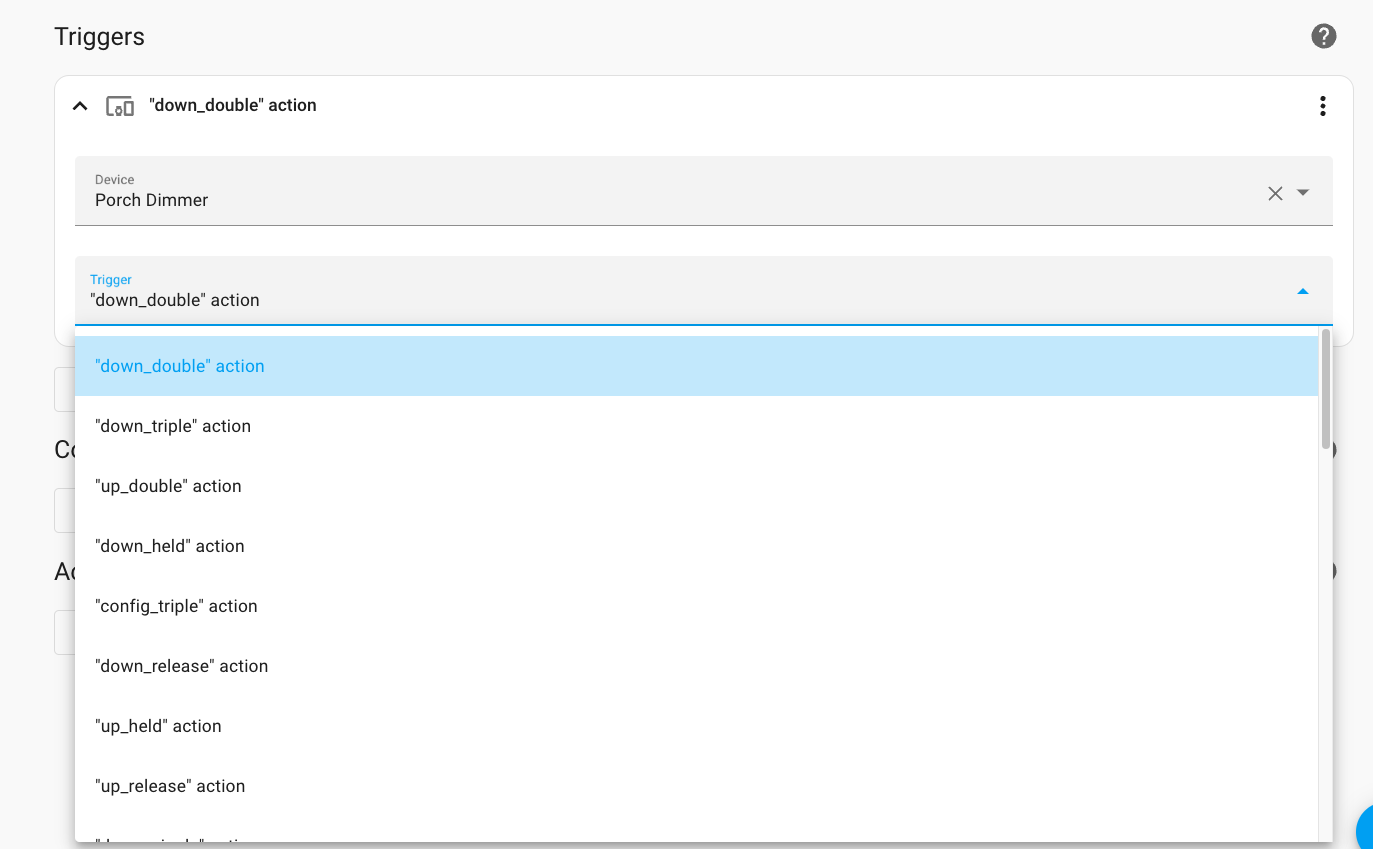This image features a detailed graphic of a device labeled "Triggers." Below this title, the text reads "Double Down - Double Action." The central component of the image is a device labeled "Porch Dimmer." Beneath the device, there is a list of various configurable options, including:

- Down Double Action
- Down Triple Action
- Up Double Action
- Down Held Action
- Config Triple Action
- Down Release Action
- Up Held Release Action

To the side of these options, the background is gray, and near the top right corner of the image, an icon in the shape of a triangle, along with a question mark, is visible.